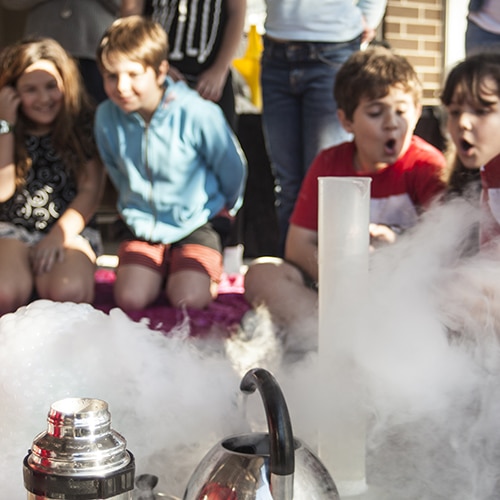This vibrant color photograph captures the excitement of four children engrossed in a science experiment. In the foreground, thick billowing smoke or steam flows from a small flask and two metal objects resembling a tea kettle and a thermos. The captivating reaction is likely caused by dry ice, sparking curiosity and amazement in the young audience. The children, kneeling on a pink blanket, showcase varied expressions of surprise and delight. On the far left, a girl smiles widely while pulling her hair back. Beside her, a child in a blue jacket and red and black shorts observes intently. To the right, two children, a boy and a girl, appear to blow towards the cloud of smoke with their lips puffed out. The background shows three partially visible adults, their upper bodies cut off by the photo's edge, hinting at their supervision. The scene exudes an atmosphere of learning and wonder, vividly demonstrating the children's engagement and joy in the scientific discovery.